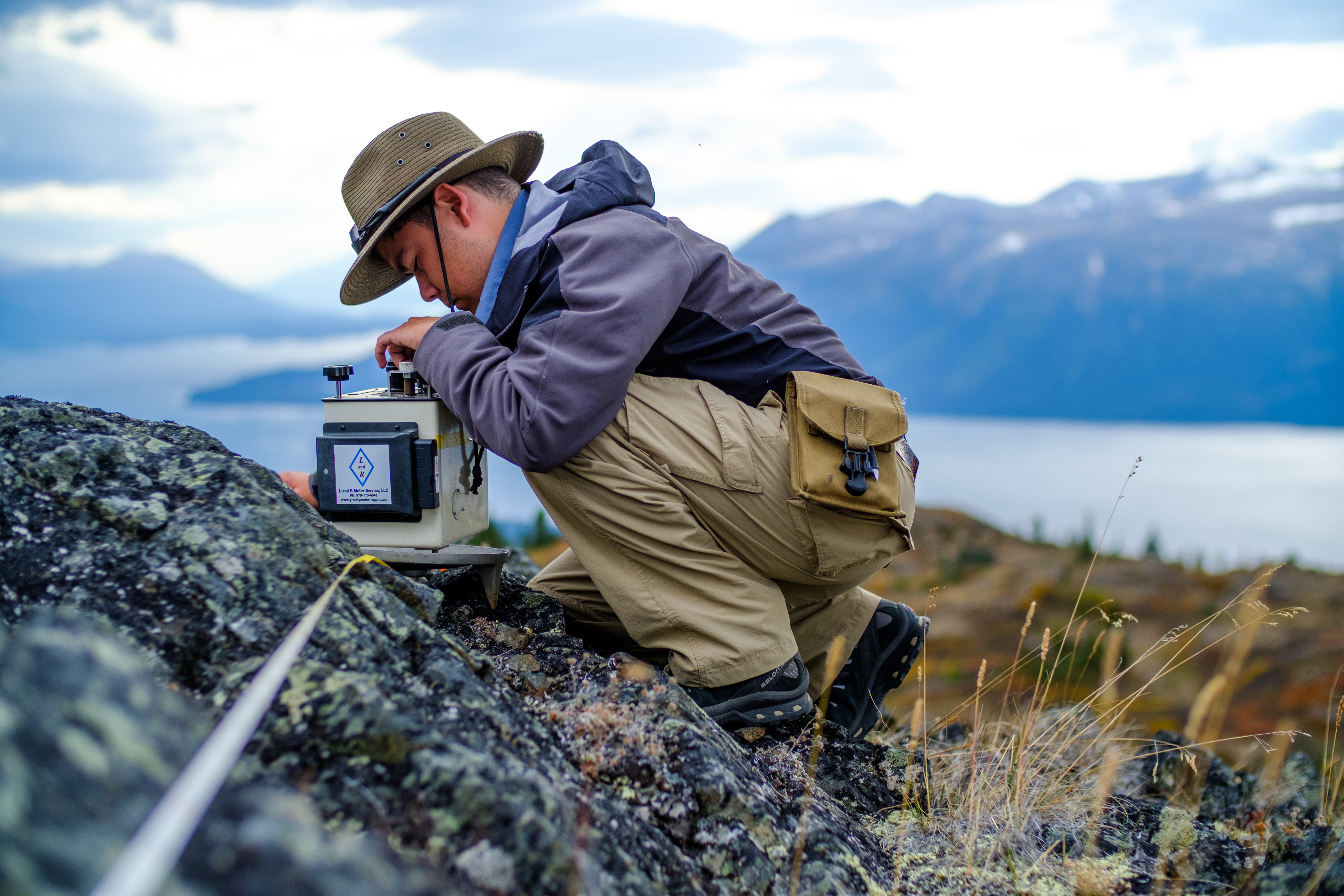A solitary man, dressed in outdoor gear including a light purple windbreaker jacket, khaki cargo pants, dark boots, and a sun-shade safari hat with a strap, is captured in an outdoor scene. He kneels on a rocky formation amidst a weed-filled field, concentrating intently on a rudimentary measurement device. This device, which features dials on top and a long wire extending from its base, is secured on a platform near his left arm. A yellow pack is attached to his belt at the back. The landscape behind him reveals a large body of water that wraps around imposing mountain ranges. The waterway curves from right-center to left-center before disappearing back to the right against a backdrop of high, rugged mountains. The sky above is a mix of clear blue and scattered white clouds, contributing to the serene yet imposing beauty of the scene. Grass and weeds surround the rocky area the man is working on, leading down to the water's edge.